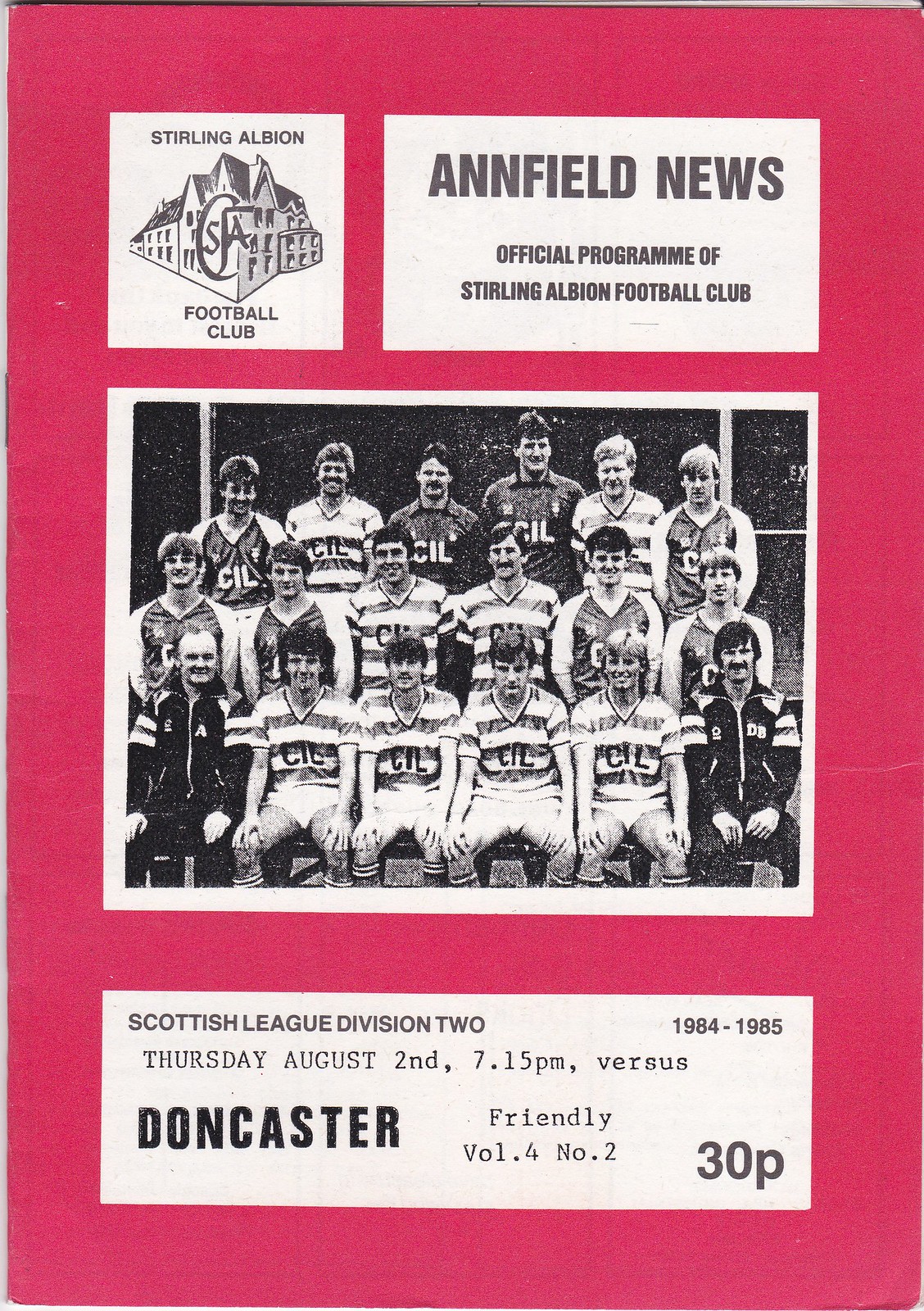This page from a magazine is the official program for the Sterling Albion Football Club, known as the Anfield News. The page has a red background and features four distinct sections. On the upper left, it prominently displays the Sterling Albion Football Club logo, with text indicating the team. The centerpiece is a black-and-white team photo of 18 men, arranged in three rows with the front row seated, and the back rows standing according to height, all dressed in striped shirts and white shorts, some wearing jackets possibly signifying their coaching roles. The photo has a grainy texture, suggesting it might be a reproduction. Below the team photo, details of an upcoming friendly match are announced: a Scottish League Division 2 game against Doncaster scheduled for Thursday, August 2nd, 1984, at 7:15 p.m. The bottom section additionally specifies that it is volume 4, number 230 of the program, priced at 30 pence.